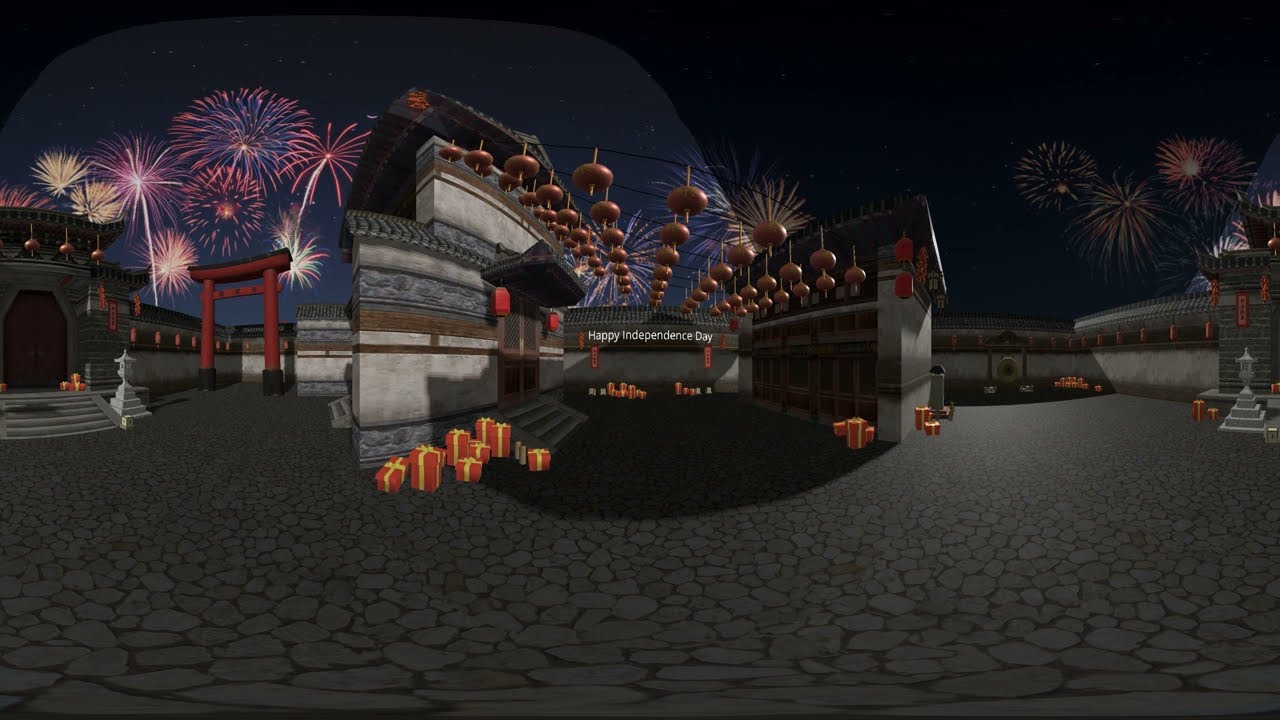The image vividly portrays a digitally rendered, animated scene, evocative of a Japanese-themed courtyard under a darkened sky illuminated by fireworks. Central to the composition is a stone-paved area flanked by traditional Asian architecture, including red lanterns and a distinctive temple entrance featuring a red arched gate. Scattered throughout are festive gifts wrapped in red with yellow ribbons. Two prominent walls frame the scene, adorned with possible Chinese symbols, although they are unreadable. Dominating the middle of the picture is white text proclaiming "Happy Independence Day." The sky above is a blend of dark blue and purple hues, providing a striking backdrop to the celebratory fireworks and enhancing the setting's festive atmosphere. Subtle details, such as a gold circular gong on the right, further enrich the intricate, immersive environment.